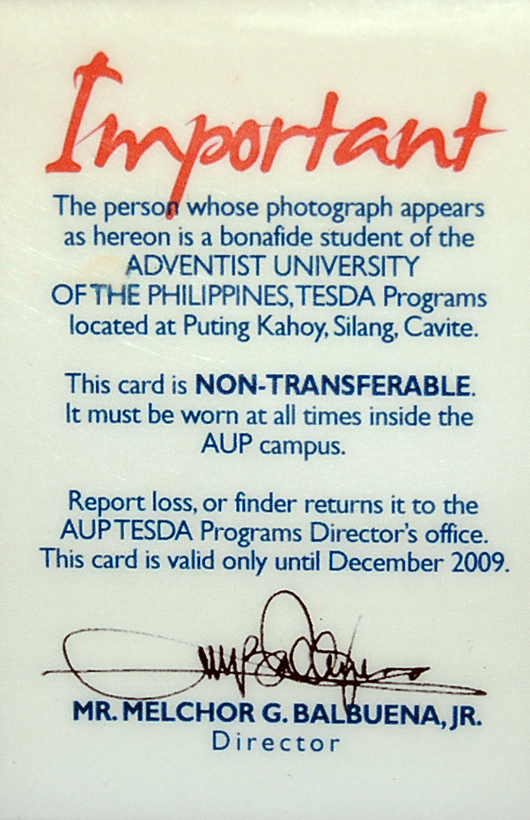This is a detailed description of an identification poster. The poster, which is white, prominently features the word "Important" across the top in bold, stylized red lettering. Below this heading, there is a section of text written in a standard blue font. It reads: "The person whose photograph appears hereon is a bona fide student of the Adventist University of the Philippines, TESDA Programs, located at Puting Kahoy, Silang, Cavite. This card is non-transferable and must be worn at all times inside the AUP campus. Report lost or found cards to the AUP TESDA Program Director's Office. This card is valid only until December 2009." At the bottom of the poster, there is a signature in black ink, accompanied by the printed name and title: "Mr. Melchor G. Balbuena Jr., Director."